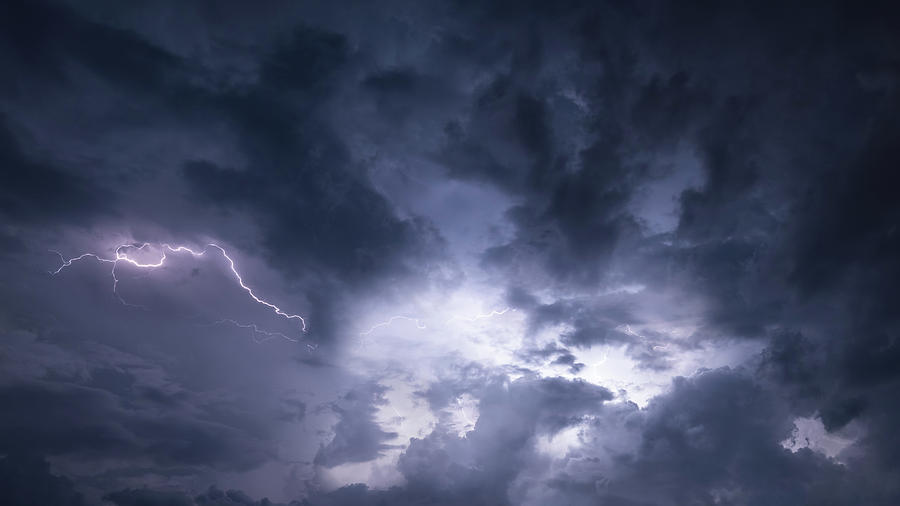In this horizontal rectangular image, a dramatic thunderstorm unfolds against a profoundly dark sky. Dominating the left side of the image, a jagged streak of lightning splits the darkness, casting a brief, intense glow. Centered and slightly to the right, a bright, almost explosive area illuminates the scene, suggesting either a powerful lightning strike or sunlight piercing through the dense, ominous clouds. This bright spot seems to light up the core of the storm momentarily before fading back into the encompassing darkness. The storm clouds, thick and foreboding, occupy most of the sky, with the darkest concentrations stretching primarily across the right side and extending towards the left. A smaller, isolated bright spot appears in the lower right corner, perhaps another burst of lightning. The overall atmosphere is charged with the chaotic and fleeting brilliance of a lightning storm amidst the oppressive gloom of the surrounding storm clouds.